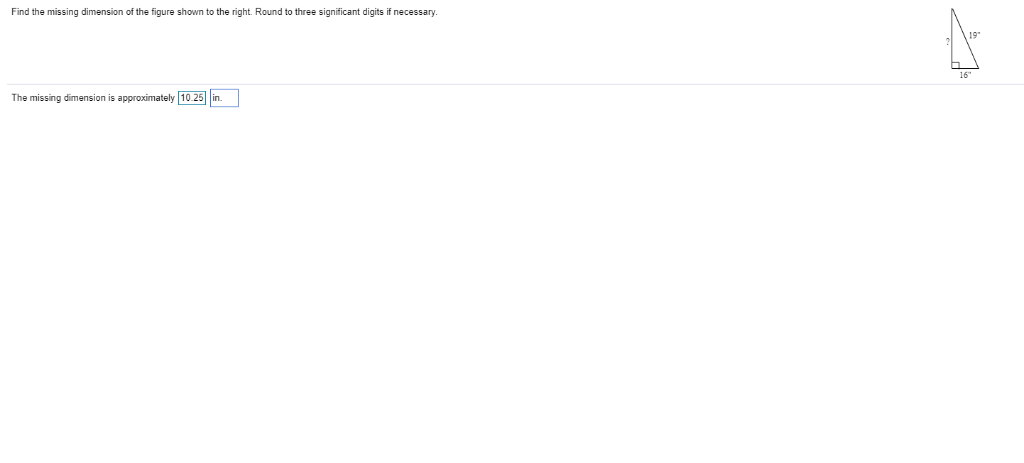The image displays a right-angled triangle against a white background, with one leg labeled as 19 inches and the other leg labeled as 16 inches. The hypotenuse, which remains unidentified, is marked with a question mark. Notably, a small square, representing the right angle, is positioned between the hypotenuse and the 16-inch side. Below this diagram, there's a turquoise-bordered box containing the calculated hypotenuse length of approximately 10.25 inches, with the unit "IN." enclosed in a separate blue-bordered box to its right. All text and lines, except for a faint gray separator line, are rendered in black, clearly dividing the instructions from the triangle illustration. The page maintains a minimalist design, with all elements aligned to the left and the triangle image occupying the right-hand side.